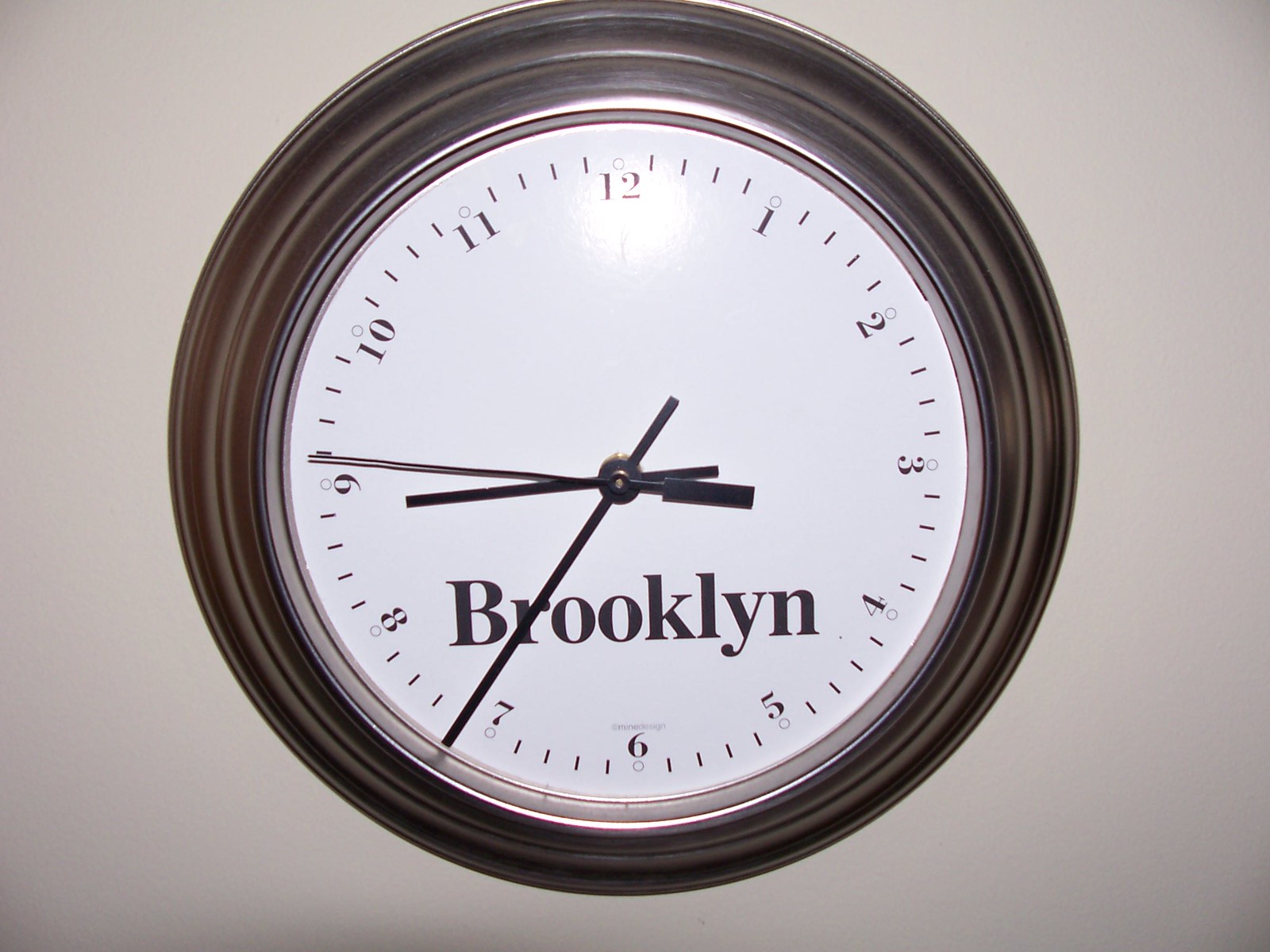The photograph captures a detailed image of a classic wall clock. The clock features a gray metal frame around a clear glass case, with a face that is bright white. The numbers on the clock are small and black, spanning from 1 to 12, with equally spaced black markings between them. Each number is surrounded by a small, black circular outline with a white center. The hands of the clock, which appear to be metal, indicate the time as approximately 8:36, with the minute hand just to the left of the seven and the hour hand slightly below the six. Additionally, the second hand is positioned just above the six. Prominently, the word "Brooklyn" is printed in bold black letters at the bottom of the clock face. The clock is set against a light gray wall, with the image background appearing a bit darker in the bottom corners. A reflection of light is visible on the top part of the clock, suggesting the photograph was taken indoors.